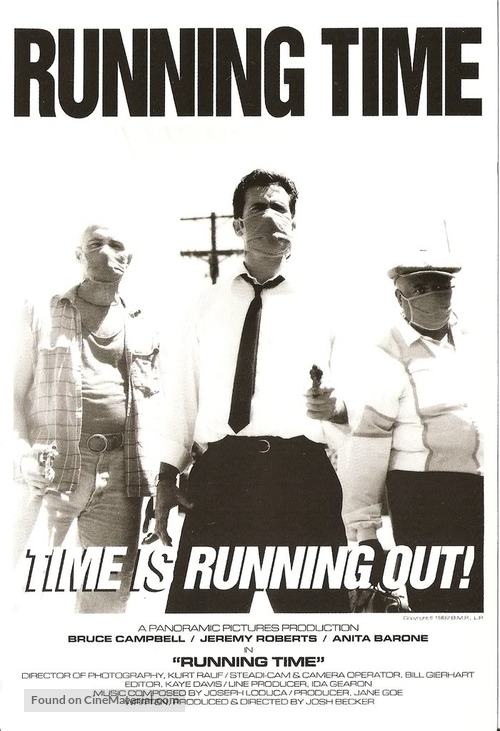The image is a black-and-white movie poster for a film titled "Running Time," displayed in bold black letters at the top. The central focus is on three masked men standing in front of a pole. The man in the center, who is holding a revolver pointed straight ahead, wears a white dress shirt with a loose black tie, dress slacks, and a black belt. He has brown hair and a medical mask covering his nose and mouth. To his left stands a man in jeans, a low-cut tank top or t-shirt, an unbuttoned flannel shirt, and a belt; he is bald and also wears a surgical mask. On the right is a man with a more casual button-up shirt, black pants, and a cap; he, too, wears a surgical mask. The bottom text prominently states, "Time is running out!" In smaller print, the poster announces it is a Panoramic Picture Production featuring Bruce Campbell, Jeremy Roberts, and Anita Behrens in "Running Time," along with additional details about the production team and associates.